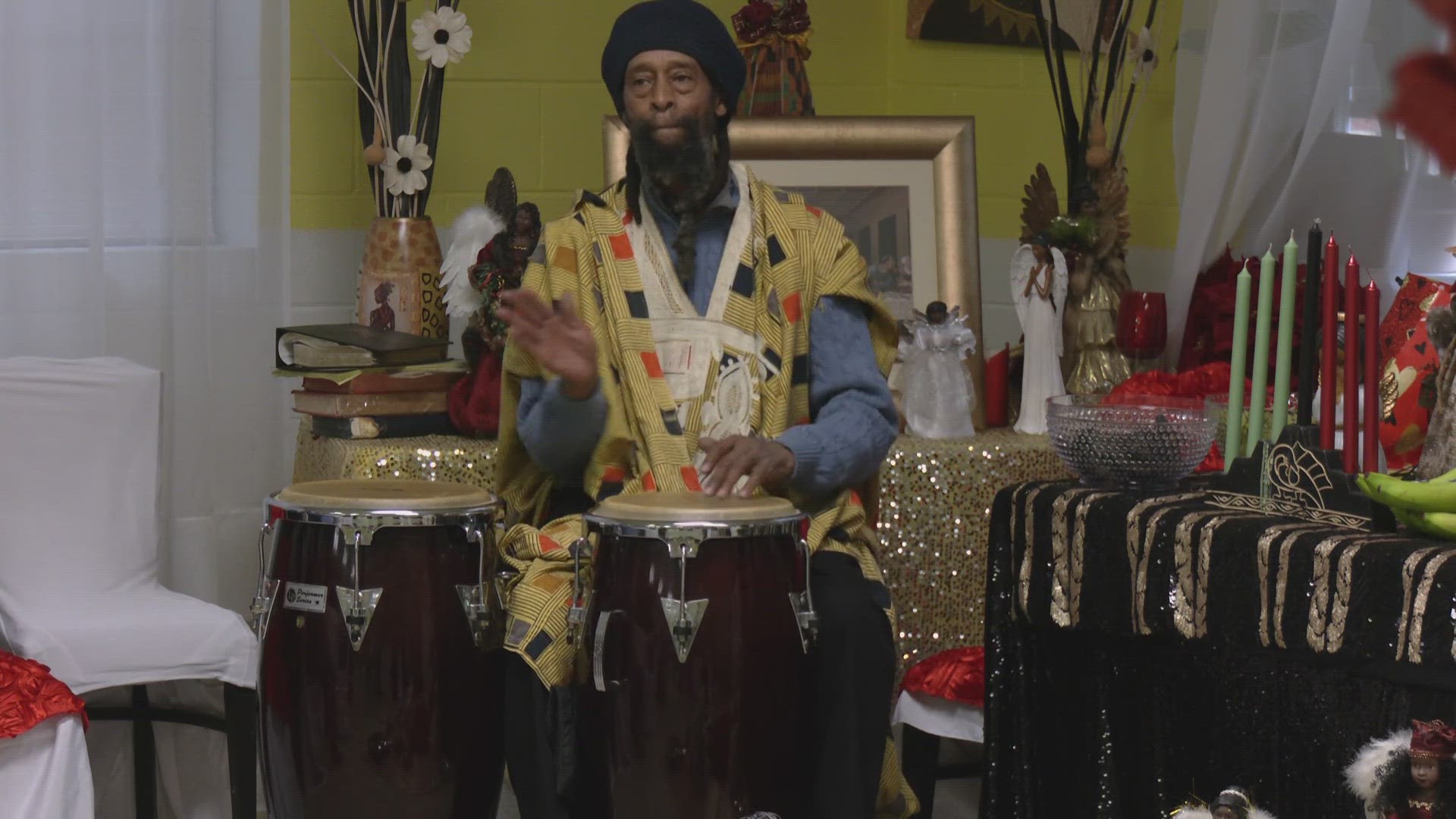In this photograph, an Afro-American man with a long braided beard and glasses is playing a bongo drum at what appears to be a religious celebration or ceremony. He is seated in a room with yellow walls and white, see-through curtains. The man is dressed in elaborate ceremonial attire, including a navy beret or turban and a vibrant African dashiki featuring yellow fabric with red and black rectangles, and a white design around the neck. In front of him are two shiny brown bongos with tan tops, although he is playing only the one positioned between his knees.

Behind the man, a table draped in a black tablecloth with golden stripes presents a candelabra arrangement featuring green, red, and one black candle, suggestive of a Kwanzaa setup. Adjacent to this is another table covered with a gold glitter tablecloth, embellished with white angel statues, flower arrangements in African vases, and some books. Additional details in the room include a chair on the left side covered by a tarp and a picture frame behind the man, flanked by flowers on both sides. The overall color palette of the photograph is somewhat dull, emphasizing the colorful ceremonial garb and table decorations.